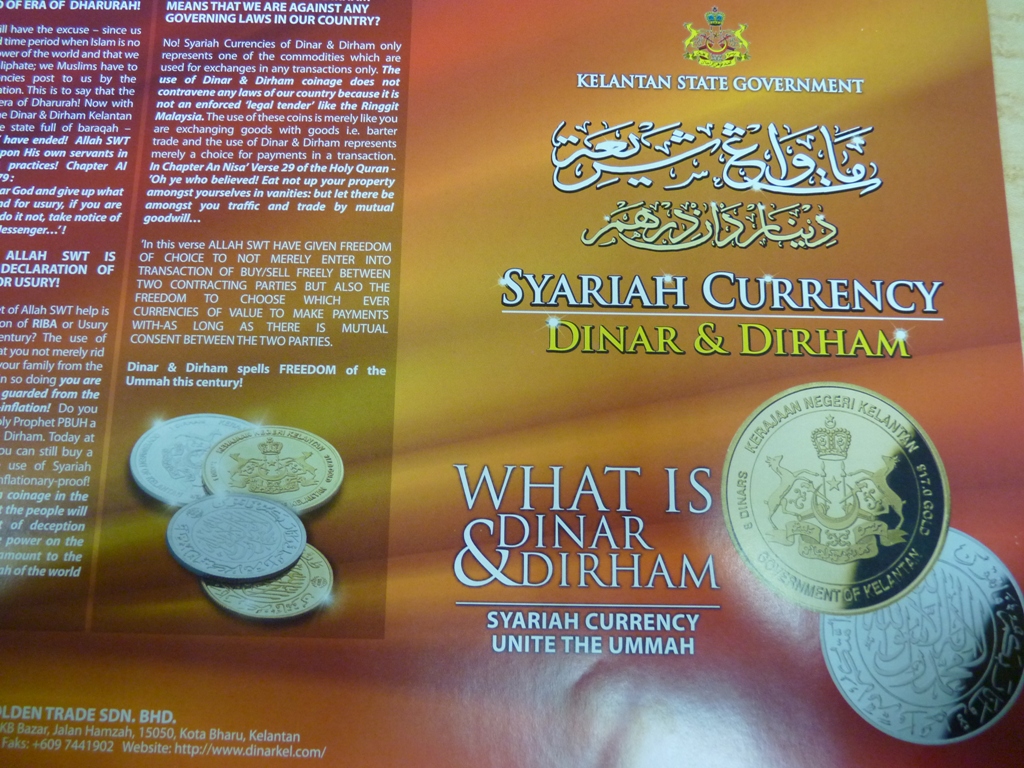The image is a detailed pamphlet page featuring a golden background with a radiating pattern. At the top, it prominently displays the Kelantan State Government logo, followed by the title "Kelantan State Government" in white. Beneath this, there are lines of text in Arabic script— the first line is in white, and the second line is in beige. Below the Arabic text, “S-Y-A-R-I-A-H currency” is underlined, with "Dinar and Durham" written in yellow. The lower section of the page highlights two coins—one gold and one silver—positioned towards the right corner, and to their left in white text it reads, “What is Dinar and Durham?” Below this, it reiterates "S-Y-A-R-I-A-H currency" and adds "Unite the U-M-M-A-H" in smaller print. The left side of the pamphlet appears to contain an illustrative column that provides a detailed explanation, mentioning that Allah SWT has given the freedom of choice to enter into transactions or buy and sell freely between contracting parties.